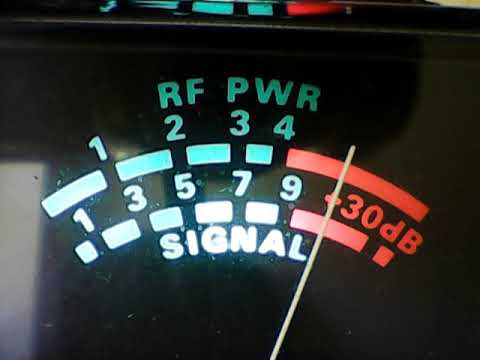The image is a detailed display gauge, likely from a device measuring amplification levels or sound output, such as from a speaker. The background is primarily black, with bold text and color accents. 

At the top of the display, "RF PWR" (short for RF Power) is prominently featured in blue letters. Below this heading, there is a semi-circular arrangement of rectangular dots, transitioning from white to blue, and culminating in a red section on the far right. These rectangles are numbered sequentially from 1 to 4.

Further down, another semi-circular array of rectangular dots appears, numbered 1, 3, 5, 7, and 9. This sequence also includes a progression from green to red, with "30 dB" (presumed to represent decibels) marked in the red area on the far right.

Beneath this second semicircle, the term "signal" is written in white. A white needle or dial extends from the center of the image, intersecting both semi-circular displays and currently pointing into the red zones of both the RF Power and Signal levels, indicating high or potentially dangerous levels.

Overall, the image is monochromatic with green and red segments to signal operational status, and no other objects are visible within the display area.